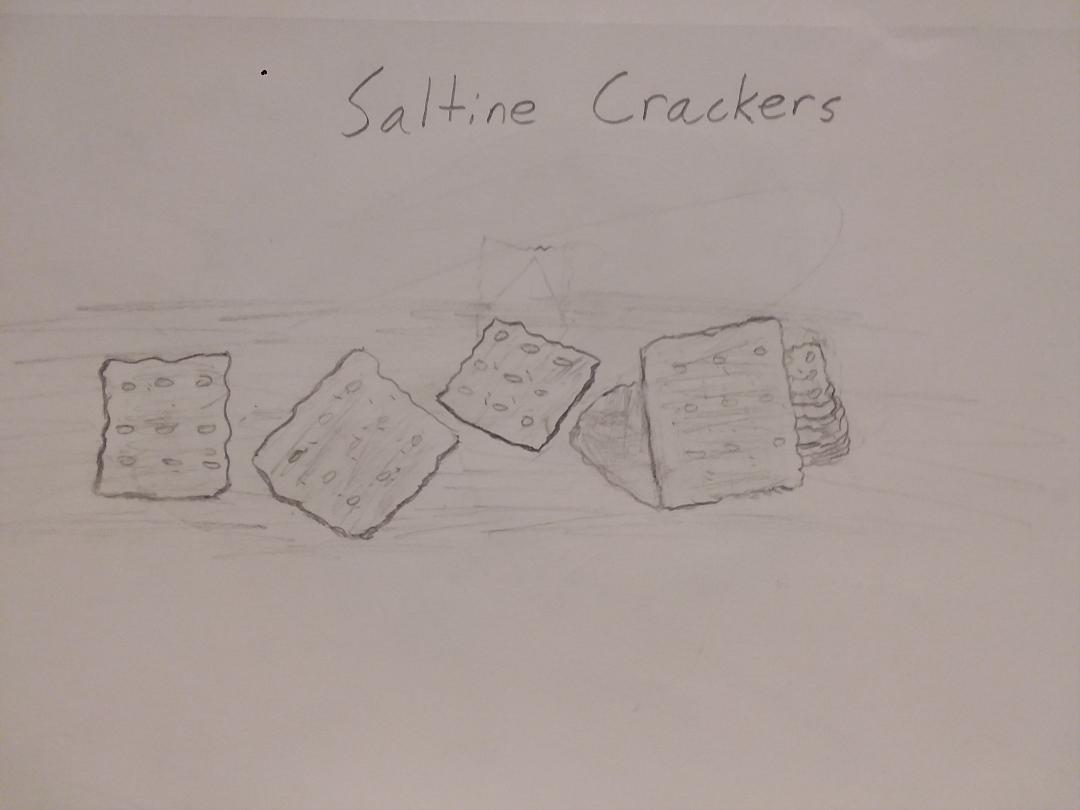A white piece of paper features intricately detailed pencil drawings centered around the theme of saltine crackers. At the top of the paper, the words "Saltine Crackers" are clearly inscribed. Just below this title, a whimsical scene unfolds: a rocket cleverly designed to resemble a saltine cracker is illustrated, complete with smaller saltine crackers as passengers hitching a ride in the back. In addition, three separate saltine crackers are depicted soaring through the air with dynamic lines indicating their movement. Each cracker is meticulously detailed with nine perforations and rugged, jagged edges. Subtle erasure marks and hints of other drawings faintly appear, suggesting underlying sketches or images drawn on the reverse side of the paper that slightly show through.